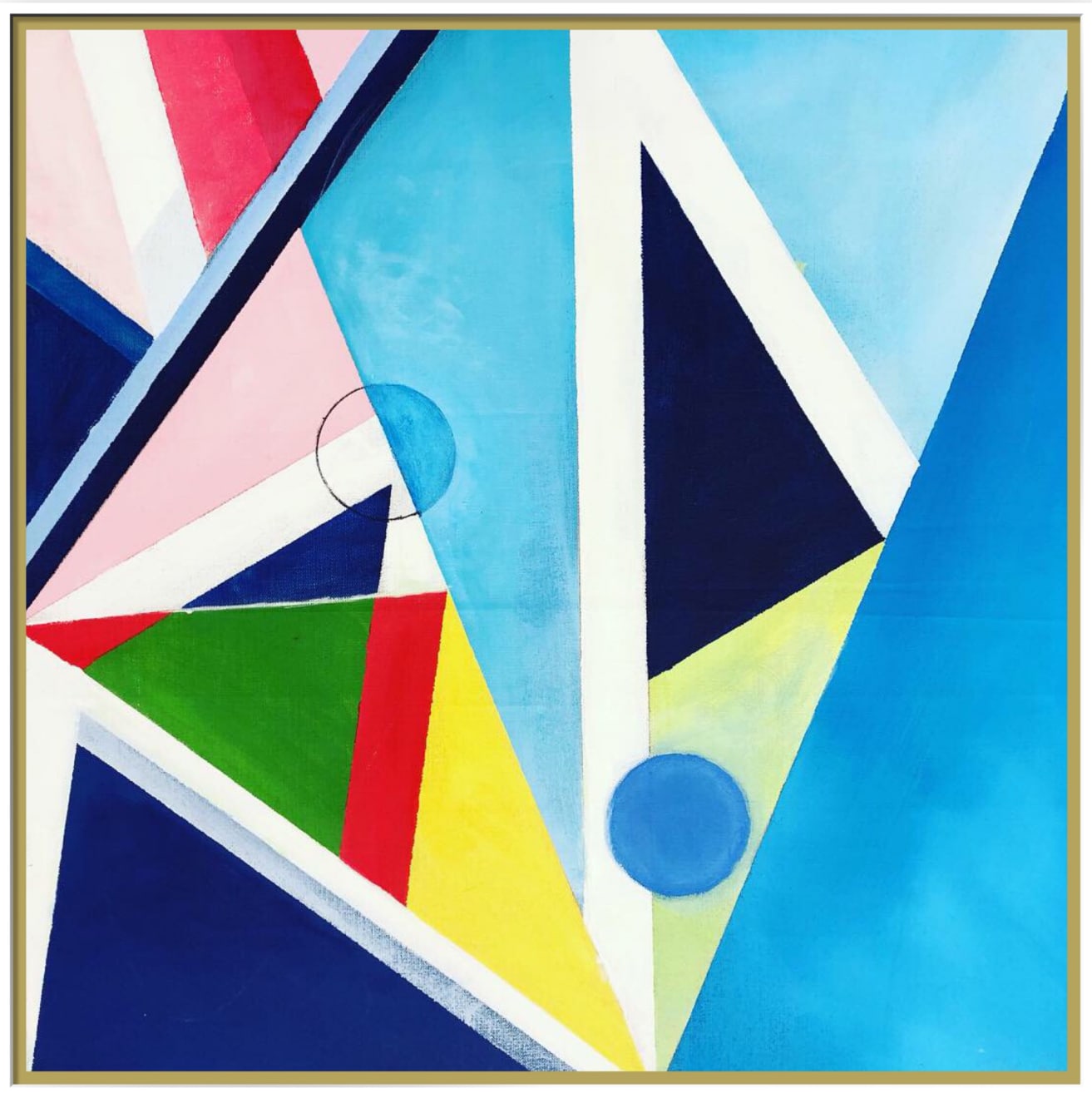This modern abstract painting features an intricate composition of various shapes, predominantly triangles, creating a dynamic and vibrant piece. The artwork is filled with a rich palette of colors, ranging from different shades of blue, green, yellow, red, white, and pink, to black. This combination of hues results in a striking contrast and depth throughout the painting. Central to the image are two circles: one is a dark or sky blue solid circle situated at the bottom, while the other, positioned on the left, is a partially filled circle with translucent elements in white, pink, and blue. The geometric shapes dominate the composition, with many triangles displaying varying sizes and angles, some reminiscent of sails on a sailboat. Despite its abstract form, the artwork exudes a vintage charm, akin to styles popular in the 1980s or early 1990s. The painting appears well-zoomed in the photograph, emphasizing its detailed and intricate design, and it is encased in a gold frame, ready to adorn a living room, office, or bedroom wall, adding brightness and artistic flair to any space.